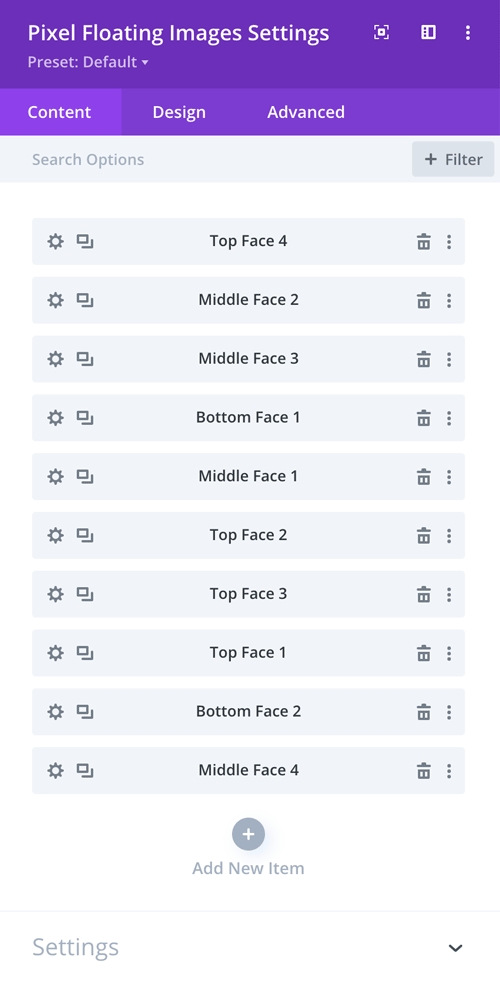The image displays a user interface on a cell phone, most likely an Android device as indicated by the "Pixel" branding at the top. The interface seems to be related to some specific settings or customization options.

At the very top, the screen title reads "Pixel Floating Images Settings," although the exact functionality of "Pixel Floating Images" is unclear. The interface title "Preset Default" is prominently displayed, accompanied by a pull-down menu that suggests options for selecting other presets.

Below the title, the screen is divided into three tabs: Content, Design, and Advanced. There is also a search filter to facilitate finding specific options within these tabs.

A detailed list of face parts follows, organized into categories labeled as top, middle, and bottom. The list includes:
- Top Face 4
- Middle Face 2
- Middle Face 3
- Bottom Face 1
- Middle Face 1
- Top Face 2

Each face part entry includes several control icons: a settings icon, a copy button, a trash can for deletion, and a three-dot menu for additional options.

At the bottom of this list, a circle with a plus sign labeled "Add New Items" allows users to add more face parts to the list.

Finally, at the very bottom of the screen, there is a settings option along with a drop-down menu indicator.

Overall, the interface looks like a detailed configuration screen for an app related to user customization, though its specific purpose remains unclear.